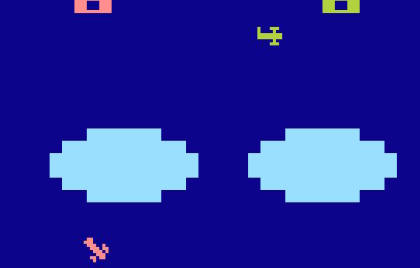The image appears to be a primitive and early-stage video game screenshot, presented in a rectangular format with a predominantly blue background. Central to the composition is a small plane, which is flying towards the right side of the screen, positioned near the center-right. The plane's design resembles a backward 'L' shape with a vertical line intersecting at the top, somewhat akin to a capital 'I' at the upper part of the 'L'.

In the upper left corner of the image, there is a partial view of a pink square, while the upper right corner displays a green square. Both these squares are contrasted with the pixelated environment. Additionally, near the center-left and center-right edges of the screen, there are pixelated, stretched, circular images that add to the retro aesthetic.

Towards the bottom of the screen, there is another pixelated object that resembles a plane. This secondary plane is angled downward, with its back end oriented towards the left side of the image. The overall composition and pixelation suggest a rudimentary graphical style typical of early video game development.